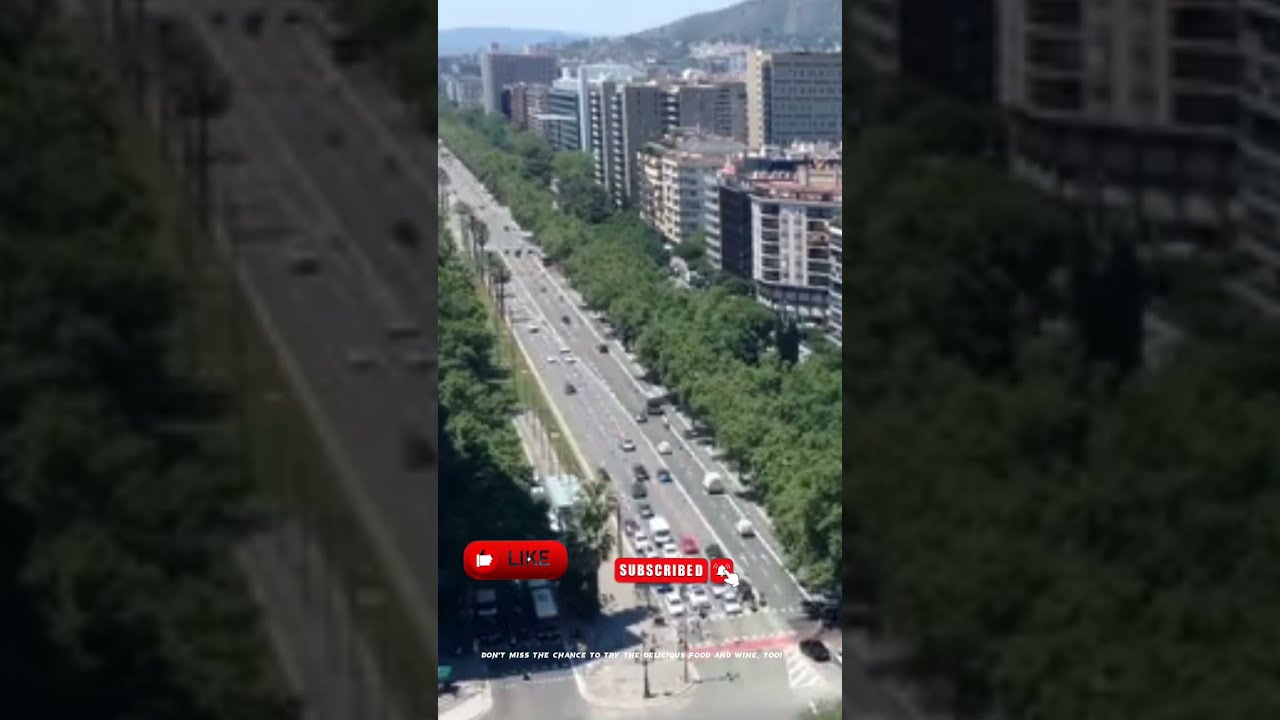The image is an aerial view of a cityscape captured from above and shared on social media, presumably YouTube. The central focus is a long, two-lane street bustling with cars, flanked by rows of verdant green trees on both sides. To the right of the trees are numerous tall buildings that appear to be hotels or office buildings, numbering around ten. The scene captures a clear blue sky framing a distant mountain at the far end of the street. Near the bottom of the image, a traffic light and pedestrian crossing are visible. Overlaying the image are familiar social media elements, including a like button, a subscribe button, and an alarm bell icon with a mouse cursor clicking on the subscribe button. The overall color palette includes greens from the trees, grays and whites from the buildings and road, and various other colors accentuating the details, suggesting an outdoor setting in the middle of the day.